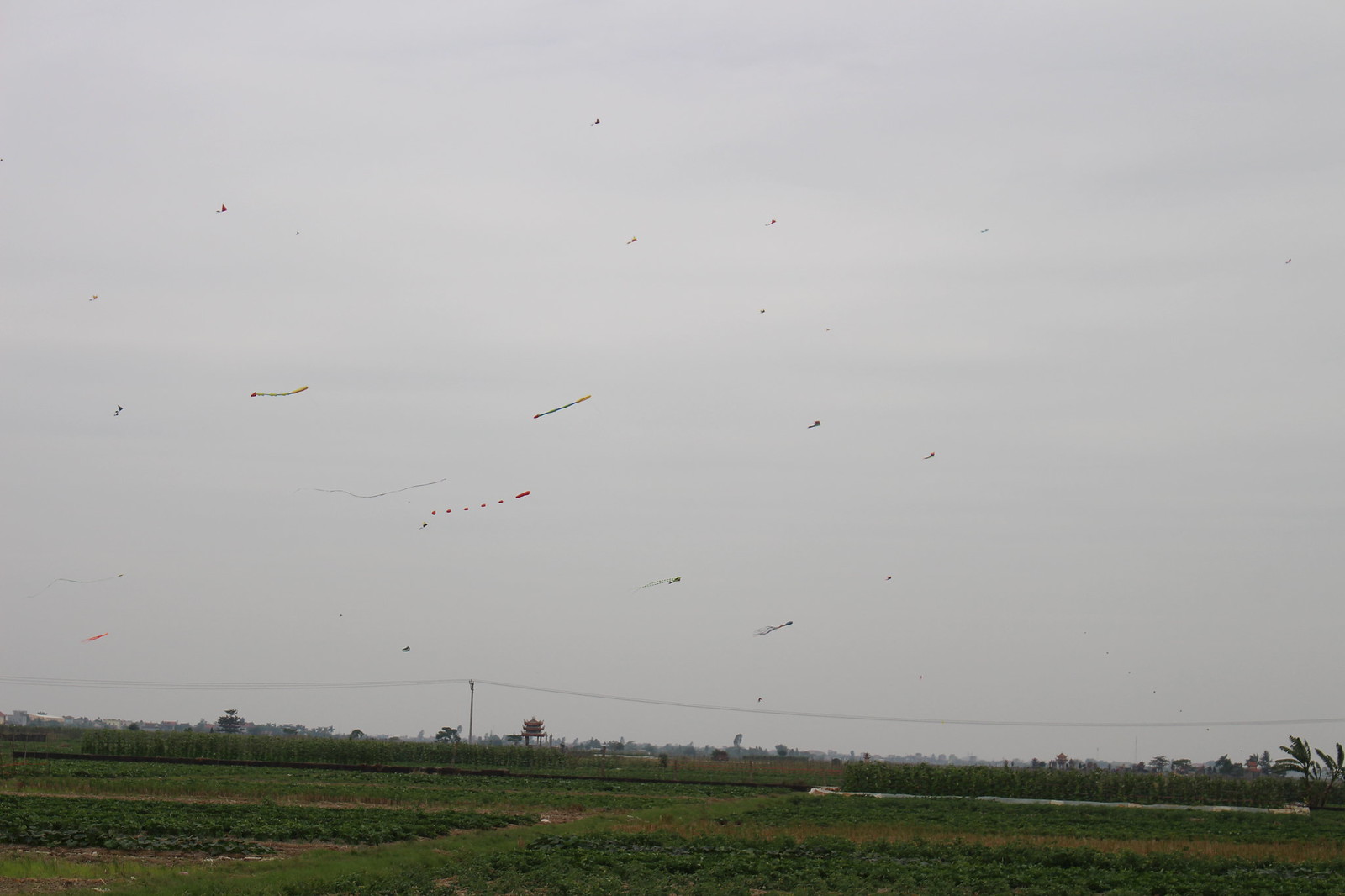This color photograph captures a large, green farm field in the foreground, characterized by rows of plowed soil and possibly growing crops. Above the field, the sky is overwhelmingly gray and overcast, occupying about 80-90% of the image. On the horizon, there is a tree line with a mix of taller trees and shrubbery, accompanied by far-off power lines and poles stretching horizontally. The most striking feature of the photo is the presence of 20 to 30 kites dotting the sky. The kites, appearing primarily as specks or thin lines with tiny tails blowing to the left due to the wind, add a dynamic yet distant aspect to the scene. The photograph seems to be taken from a considerable distance, making it difficult to discern the kites' colors and finer details, and no people are visible. Overall, this image evokes a sense of quiet, solitary activity under a foreboding, gray sky.